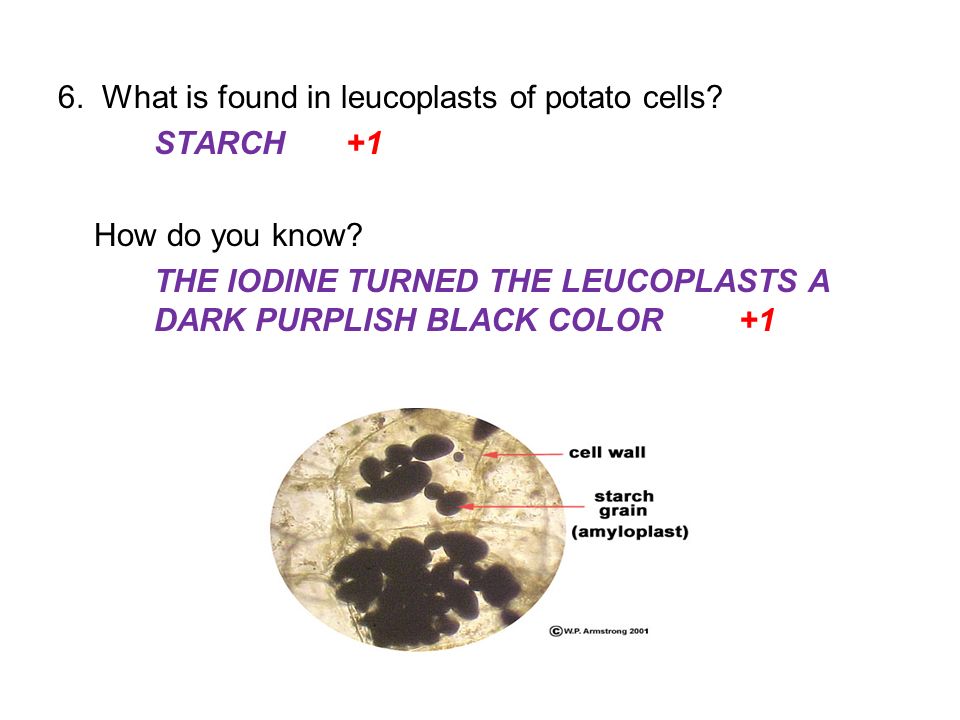The image depicts a biology-themed PowerPoint slide or textbook page against a white background, illustrated with questions and answers regarding leukoplasts in potato cells. At the top, in black text, is the label "6. What is found in leukoplasts of potato cells?", followed by a response in purple text, "STARCH", and a red "plus one". Below it, another question in black text asks, "How do you know?", accompanied by the answer in purple, "The iodine turns the leukoplasts a dark purplish-black color", with another red "plus one". The slide also features a detailed microscopic image at the bottom. This image shows a cross-section of a cell with a red arrow pointing to the cell wall labeled in black. Smaller red arrows indicate "starch grains," with a corresponding label in black that includes the term "amyloplast" in parentheses. This elaborate illustration is accompanied by a citation below, "Copyright WP Armstrong 2001".